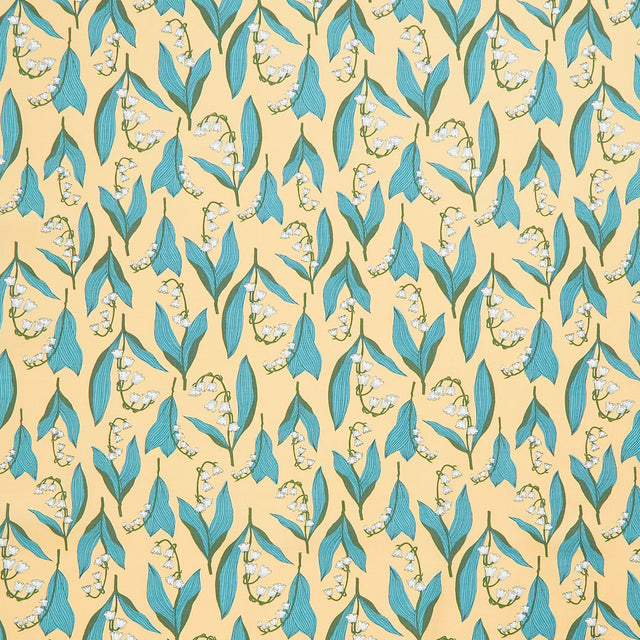The image portrays a seamless, repetitive pattern with a pale yellow, almost tannish background. This square-shaped design features delicate, green stems resembling thin spaghetti noodles, curving gracefully like candy canes. Each stem supports two teal and dark green leaves, sometimes appearing as a single leaf at a quick glance. The leaves are either closer together or slightly spread apart, creating subtle variations within the pattern. Adorning these stems are small, white, bell-shaped flowers, ranging from five to nine per stem. Some of these floral arrangements appear upright while others hang upside down, adding a dynamic sense of movement to the design. The overall aesthetic is reminiscent of a wallpaper, with no text or people, just intricate drawings repeating across the entire background.